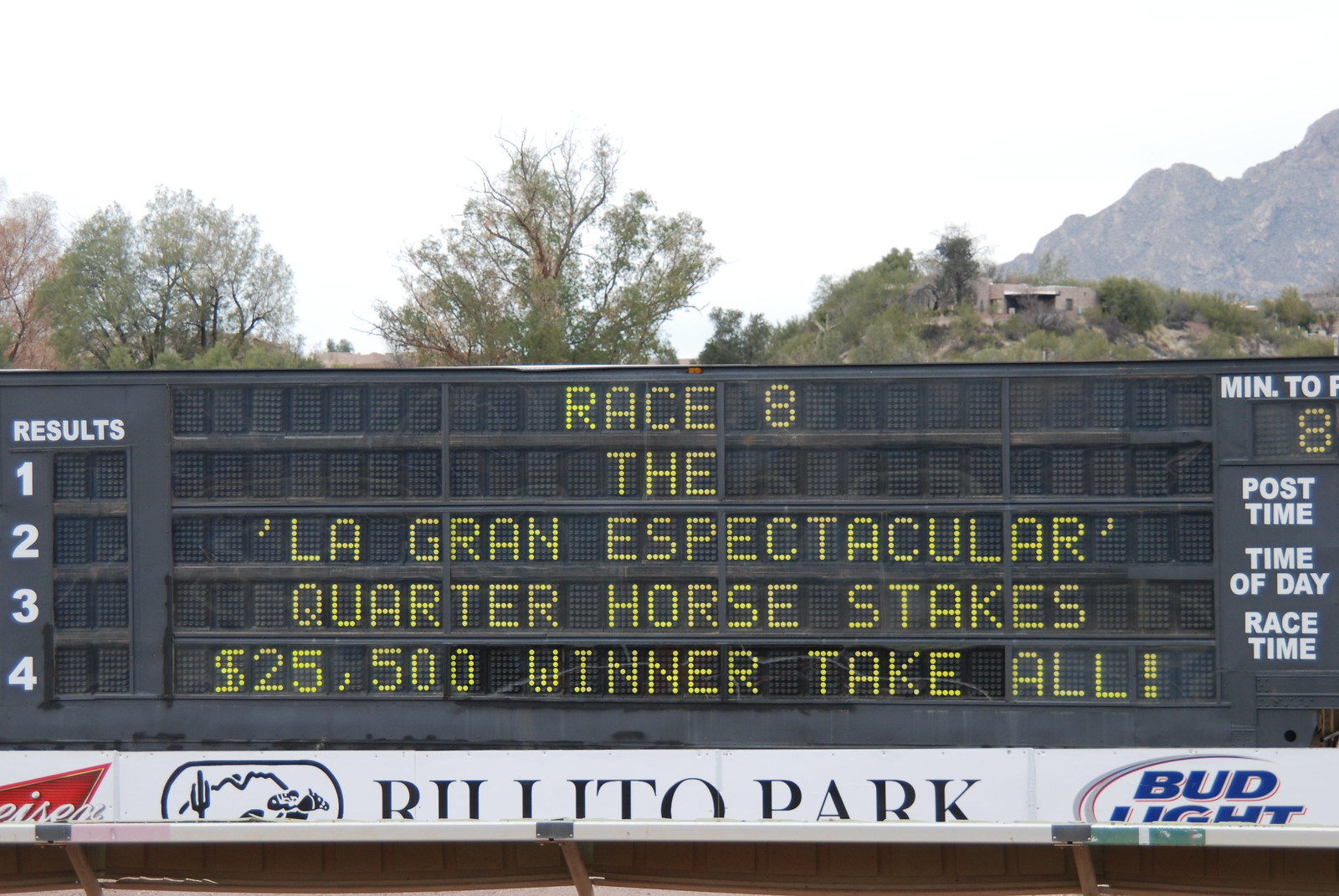The image features a detailed scoreboard from a horse racing event at Bolitoe Park, prominently displaying information for Race 8, the La Grande Spectacular Quarter Horse Stakes, with a $25,500 winner-take-all prize. The scoreboard, characterized by yellow text composed of small squares against a black background, details race results sections, which currently show "1, 2, 3, 4" on the left, and "Minute to Post: 8" on the right, along with placeholders for post time, time of day, and race time. At the bottom of the scoreboard, there are advertisements for Budweiser on the left and Bud Light on the right. Additionally, a logo depicting a man on a horse next to a cactus is displayed. In the background, the scene is set against a backdrop of mountains, trees, and a cloudy, white sky.